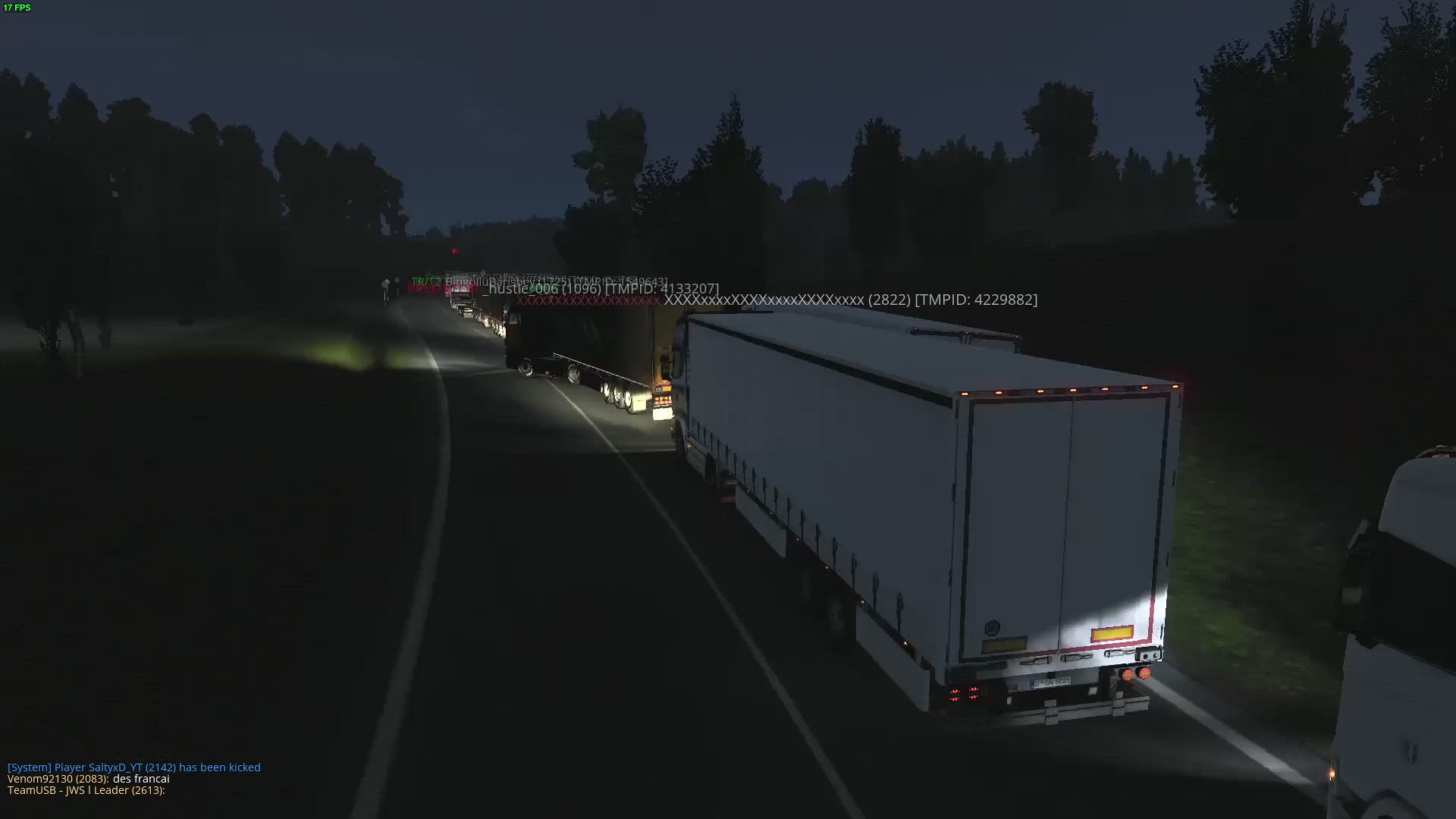This horizontal, rectangular color photograph, likely a still from a video game, depicts a serene yet eerie nighttime or twilight scene on a two-lane road flanked by dark forests. The road, marked by a single white dashed line down the middle, extends into the distance, disappearing into the gloom. A procession of semitrailers dominates the right lane, starting from the bottom right corner to recede into the background. Prominently in the middle of the frame, there are two white lorries followed by a black one, with possible additional vehicles farther back. Above each truck, white text strings consisting of letters, numbers, and symbols float, suggesting a digital overlay, typical in video game interfaces. The dark sky above is tinged with dark blue, enhancing the atmosphere. The lower left corner features three lines of text: the first in blue and the next two in a creamy color, with phrases like "system," "player," "has been kicked," and "leader," indicating usernames and statuses consistent with an in-game display. This comprehensive scene skillfully blends the mundane with the digital, evoking a sense of a digital forest roadway at the brink of nightfall.